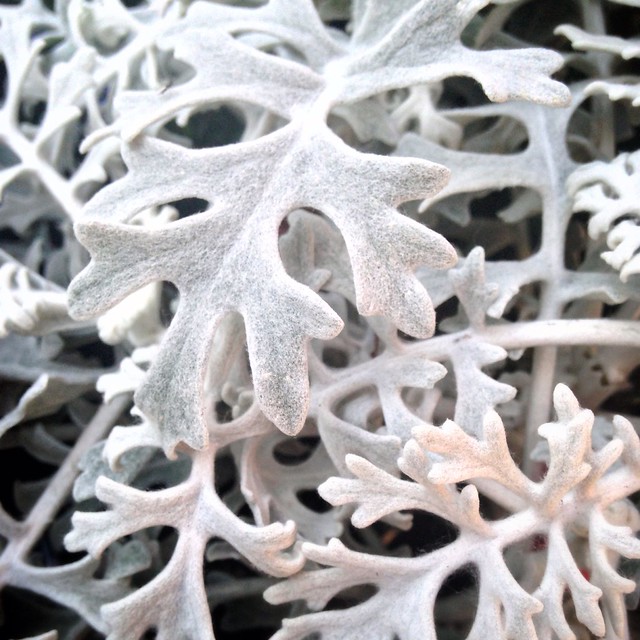The image captures a close-up of a plant with intricately detailed, frosted white leaves, likely Silver Dust. The plant features long stems from which leaves emerge. Each stem tip expands into a central longer leaf flanked by smaller leaves on either side. The leaves, some of which appear to have something like "fingers" extending outward, come in various sizes and densely cover the entire view. The scene might be taken outdoors or in a potted setting, with a contrasting black background that accentuates the stunning white foliage. The white coloration could be natural or possibly due to snow, frost, or even a spray-painted effect.